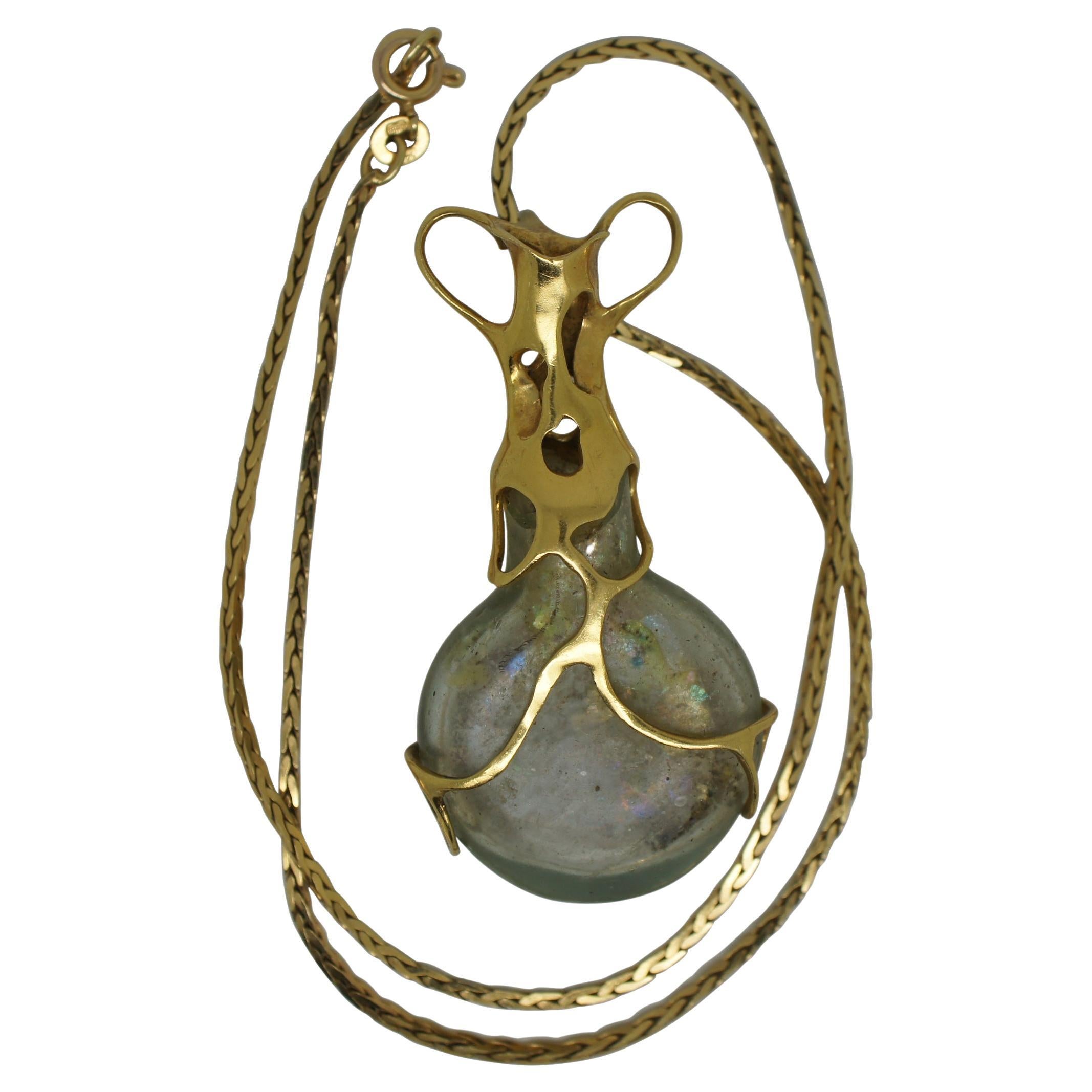The image shows a unique, vintage-style necklace featuring a gold braided chain. The chain is clasped together and elegantly curves from the top left, looping around to the bottom, then extends up to the right middle before attaching to an ornate pendant. The pendant is adorned with two large loops at the top, suggesting an antique design. The central piece of the pendant is a round, grayish-brown stone, which appears more matte than shiny, encased in a gold or bronze frame. The gold frame secures the stone with intricate lines or sections, giving the entire necklace a distinguished and timeless appearance against a white background.